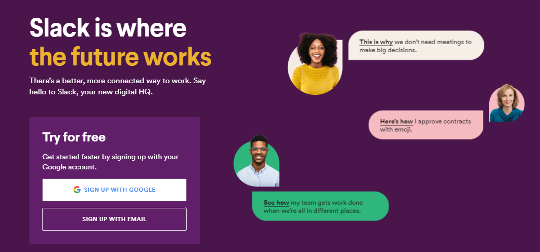Slack Homepage Description:

The homepage of the Slack website features a sleek, dark purple background. Dominating the upper left corner is the headline in the largest font, proclaiming "Slack is where the future works." Directly beneath this tagline, there is a slightly lighter purple button with the text "Try for free," accompanied by links for signing up with email or Google.

On the right side of the page, three speech bubbles display testimonials from Slack users, each featuring a portrait. The top bubble showcases a Black woman wearing a yellow shirt with a white background. Below, another bubble features a White woman in a blue shirt set against a pink background. The final bubble presents a Black man with a green background. Each portrait adds a touch of personalization and variety to the page, highlighting the diverse community that uses Slack.